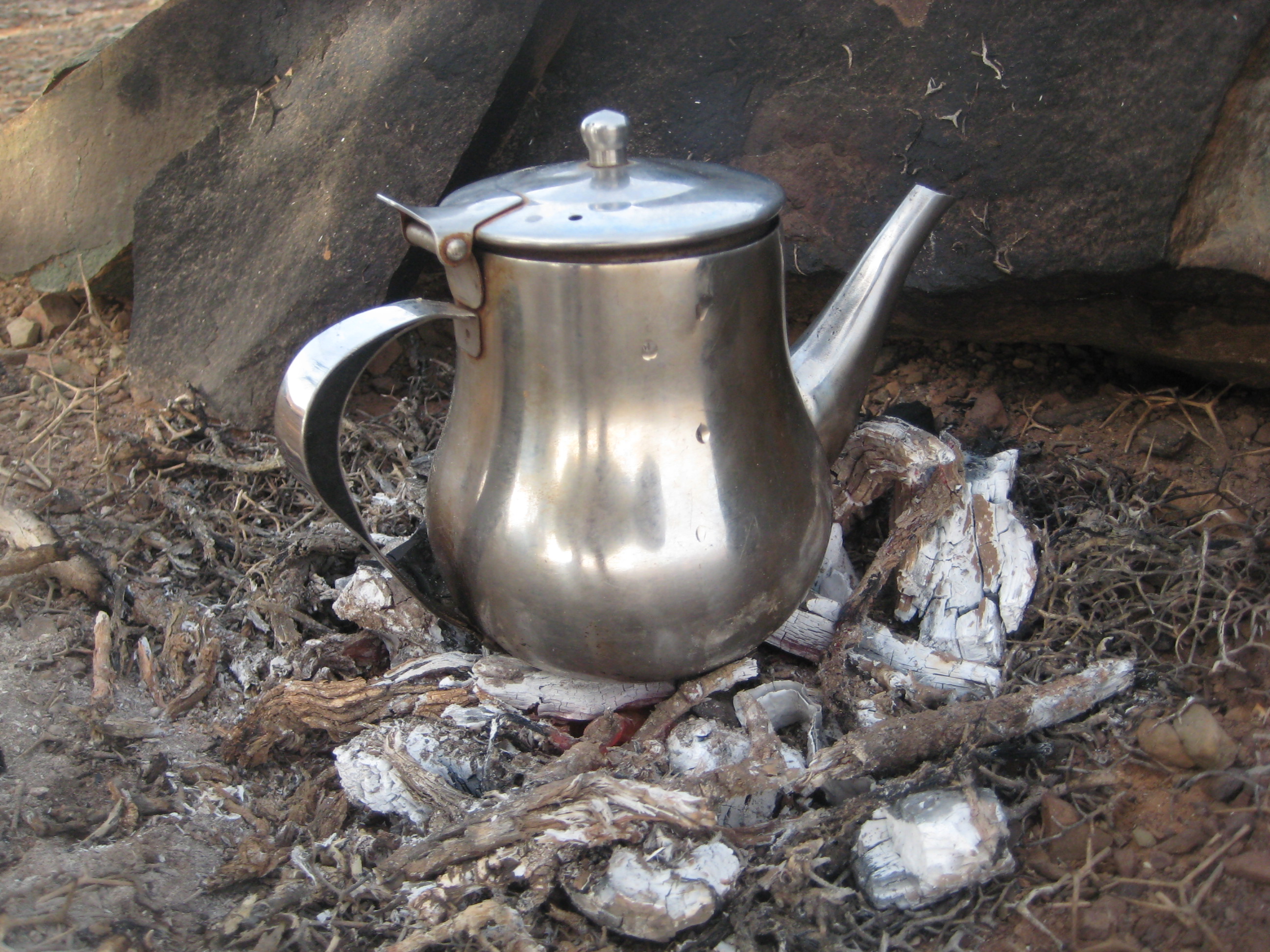In this outdoor scene, a sturdy, steel camping kettle or coffee pot rests directly atop a small, controlled fire comprised of both charcoal and wood. The flames flicker modestly at the foot of imposing gray and brown boulders. The charcoal briquettes have mostly turned to ash, intermingling with a few wooden sticks. Positioned in this rocky, relatively safe environment, the kettle stands out with its pitcher-like shape, complete with a handle and a spout. The handle, situated on the left, curves gracefully over the kettle, leading to a hinged lid that can be flipped open. The surface of the kettle is slightly weathered, possibly from minor dents or droplets of water. Surrounding the fire are patches of dry grass, though the primary setting consists of rocks and ash, ensuring a mindful and secure campfire setup.